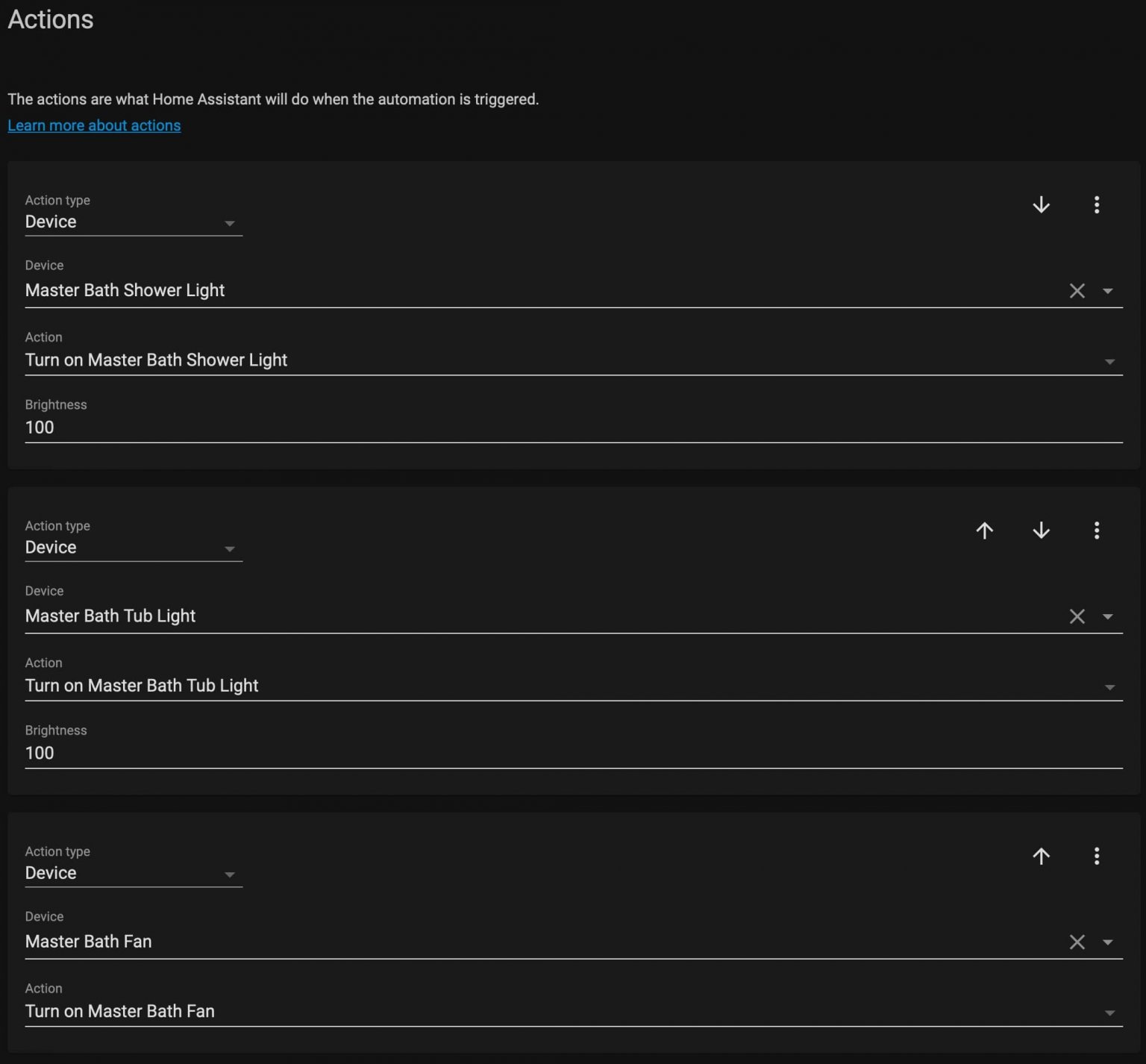In this detailed image of a device settings page, predominantly set against a solid black background, we observe a configuration screen for an automation system, likely Home Assistant. 

At the top left corner, there's the word "Actions" in bold, white text. Directly underneath it, a brief description in white reads: "The actions are what Home Assistant will do when the automation is triggered." Below this, in blue text acting as a hyperlink, it says "Learn more about actions," with a thin blue line underscoring it.

The image is divided into three distinct rectangular sections, each on a slightly lighter black background, and separated by thin white lines. 

The first section details the following:
- **Action Type**: The category of the action.
- **Device**: Lists "Master Bath Shower Lights."
- **Action**: Specifies "Turn on Master Bath Shower Lights."
- **Brightness**: Set to "100."

The second section mirrors the first but pertains to a different device:
- **Action Type**: Identical to the first section.
- **Device**: Lists "Master Bath Tub Light."
- **Action**: Specifies "Turn on Master Bath Tub Light."
- **Brightness**: Set to "100."

The third and final section, located at the bottom left, includes:
- **Action Type**: As consistent as the previous sections.
- **Device**: Lists "Master Bath Fan."
- **Action**: Specifies "Turn on Master Bath Fan."

This well-organized layout indicates a systematic approach to configuring multiple devices within the master bathroom, each with a clearly defined action and, when applicable, brightness level settings.